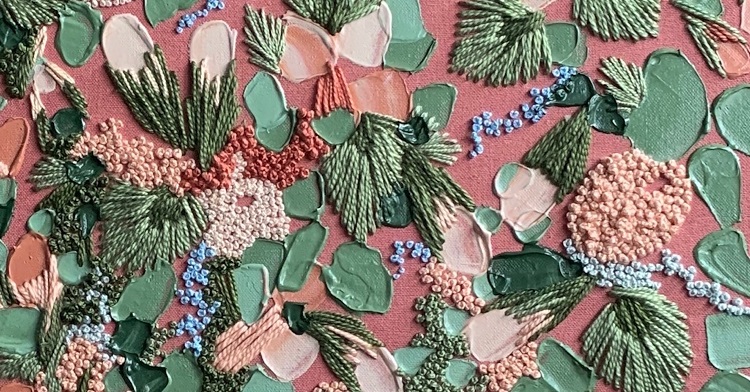This image depicts a vibrant, textured artwork on a pink or mauve fabric backdrop. The composition features an array of multicolored elements, including dark and light green yarn strands mimicking the appearance of wheat. Spread across the canvas are various shades of pink, from carnation to hot pink, and hues of blue and salmon. Intermixed with the yarn are small, circular beads in blue, white, and tan, resembling an array of tiny fruits or plant elements. Additionally, the artwork includes stitching work, with embroidered leaves and petals in different styles and colors, such as blue and green. Adding to the intricate design are tiny, popcorn-like textile pieces, wax blobs in seafoam green and pink, and elements of brocade or yarned stitchings, forming an overall dense and lively visual display. This piece could represent a rich tapestry of intertwining nature-inspired motifs, possibly suggesting a theme of botanicals crafted through mixed media.